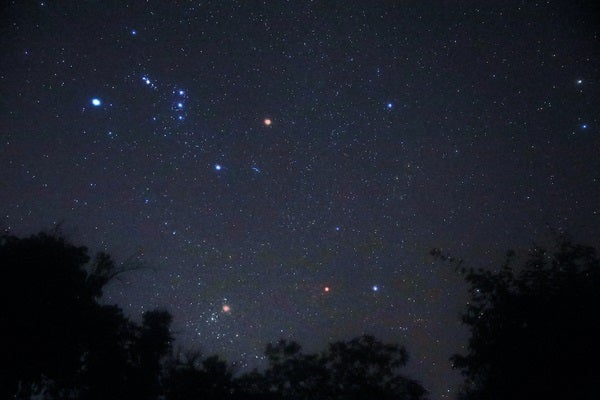A breathtaking photograph of the night sky showcases a dense carpet of stars, each appearing magnified against the dark, almost steel-gray backdrop. Orion's Belt is distinctly visible in the upper left corner, its iconic three-star alignment glowing brightly. Two notable stars emanate intense hues, with a blue star shimmering prominently in the top left and a red star radiating near the center. Scattered throughout the sky, tiny pinpricks of light create a stunning tapestry of blue and red orbs. The bottom edge of the image is framed by the silhouettes of feathery trees, adding a sense of scale and depth to the expansive celestial scene. The exposure and lighting have been meticulously adjusted to amplify the visibility of thousands of stars, making the sky appear almost alive with their glow.